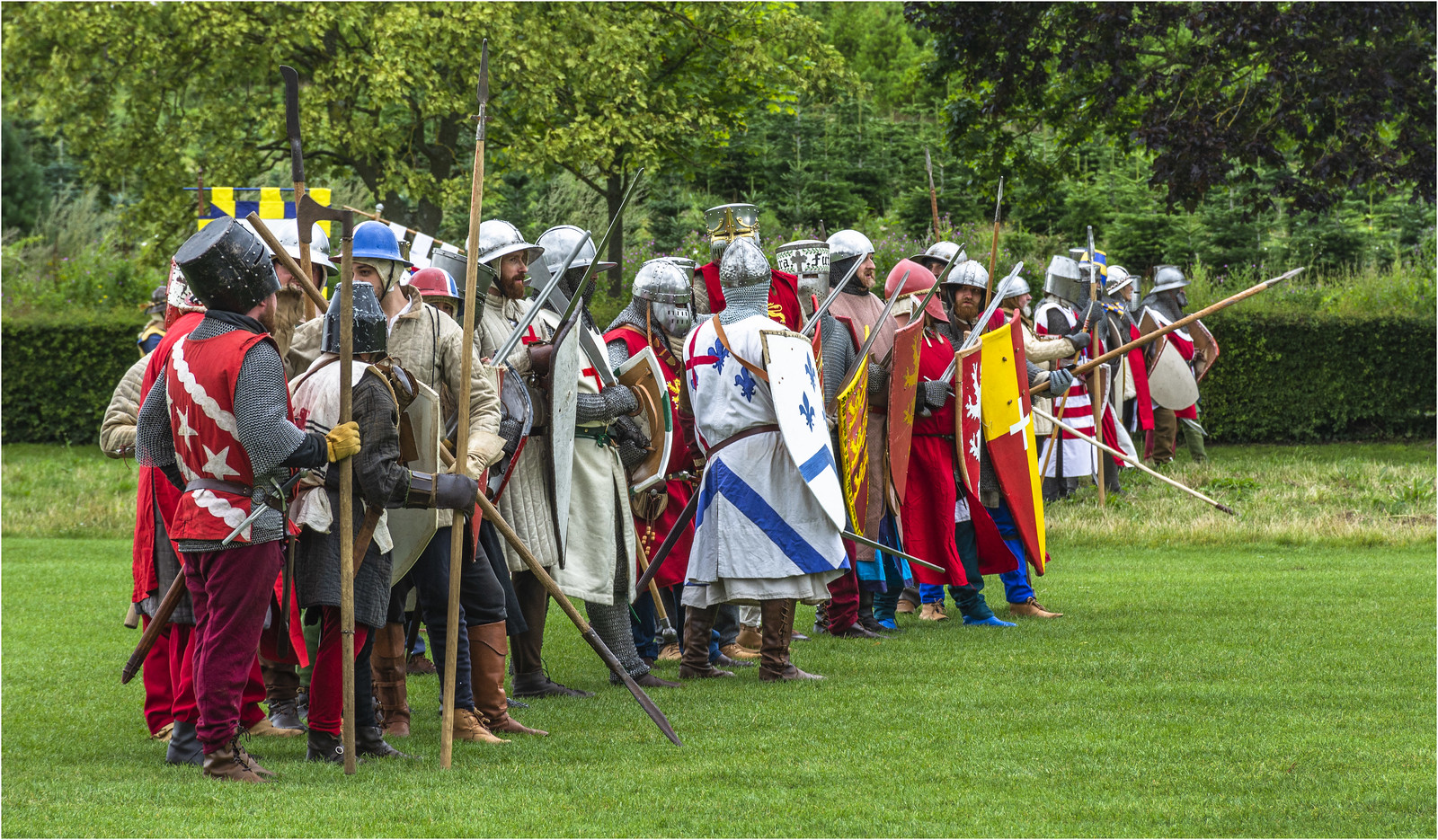In this outdoor photograph, a diverse group of men of varying ages dressed in medieval and ancient costume attire is gathered on a lush, green lawn. They stand in a slightly disordered line that stretches from the lower left corner to the center right of the image, in front of a backdrop of vivid green trees. The men's outfits include an array of colorful garments, featuring shades of white, blue, red, yellow, and gray, with designs ranging from Roman soldiers to Knights Templar and gladiators. Many are outfitted with metal helmets in different styles and colors, such as silver, black, and red, while some wear other types of hats. Their equipment includes wooden spears, shields, and various types of staffs or swords. The scene is lively and detailed, evocative of a historical war reenactment. The beautifully groomed grass and the vibrant costumes add to the visual richness of the image.